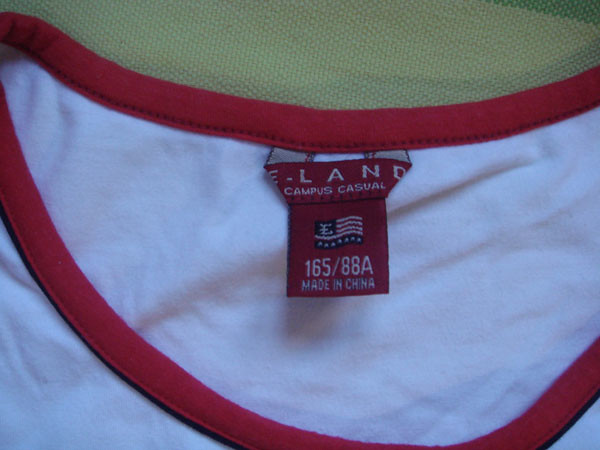This detailed photograph captures a close-up of a label on a garment, likely a crew neck shirt. The shirt is laid out on a green surface. The label displays the size "165/88A" and indicates that it is "Made in China." Additionally, the brand name "Campus Casual" is visible, along with part of the word "Land" (L-A-N-D), though the rest is obscured by a fold in the label. Notably, a red stripe is visible at the top of the label. The image suggests the garment is made from a soft, knit fabric, characteristic of a crew neck shirt, rather than the elastic material typical of underwear. The shirt itself appears to be white.